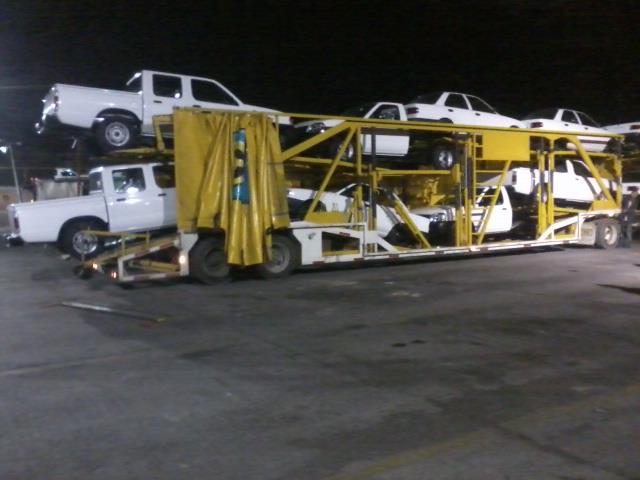The image depicts a dimly lit parking lot, likely at a truck stop, with a semi-trailer truck equipped to haul multiple vehicles. The ground is gray and marked with parking lines. The semi-trailer is enclosed with a yellow curtain, which is partially pulled back, offering a glimpse of an emblem that remains obscured. The trailer is loaded with several white vehicles, predominantly four-door trucks, although a few single-cab trucks are also seen. The vehicles are stacked in an organized, yet somewhat congested manner, with two of the trucks positioned diagonally, appearing to hang slightly off the left side of the trailer. These trucks are securely fastened for transport, either to or from a car dealership. The overall scene combines elements of industrial transport with the meticulous arrangement of new vehicles, poised for delivery.